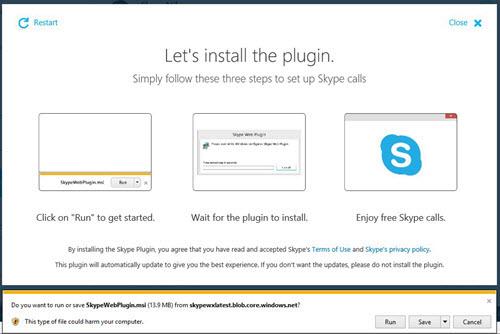In the top left corner of the image, there is a blue circular arrow icon adjacent to the word "restart." On the opposite side, the word "close" appears in blue, next to an "X" icon. The center of the image prominently displays the message "Let's install the plug-in," followed by instructions in black text: "Simply follow these three steps to set up Skype calls."

Below these instructions are three numbered squares:

1. Under the first square, the text reads: "Click on 'Run' to get started."
2. The second square instructs: "Wait for the plug-in to install."
3. Inside the third square is a blue circle with a white "S" in the middle. Below it, the text says: "Enjoy free Skype calls."

A disclaimer at the bottom reads: "By installing the Skype plug-in, you agree that you have read and accepted Skype's Terms of Use and Skype's Privacy Policy."

Beneath a long black line and a yellow line is a prompt: "Do you want to Run or Save Skype Web plug-in?" It also includes a warning: "This type of file could harm your computer," accompanied by an image of a black shield with a yellow outline. To the right, three gray buttons offer the choices: "Run," "Save," or "Cancel."